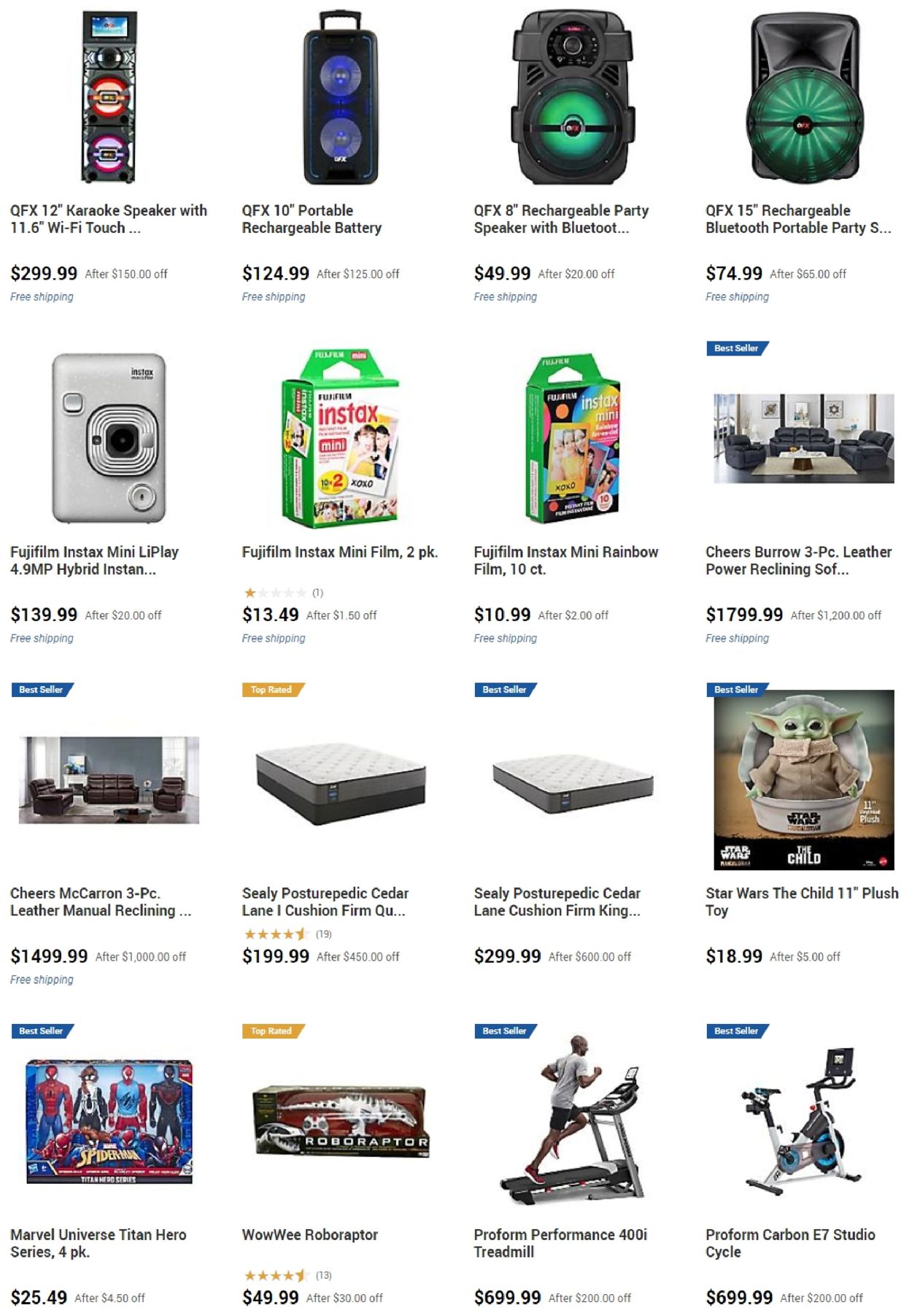The image displays an array of products organized in rows. 

On the first row:
- A karaoke speaker with a striking red and purple design priced at $299.99, featuring an 11.6" Wi-Fi touch screen.
- To its right, a vertical blue speaker priced at $124.99.
- Next, a green speaker priced at $49.99.
- Another green speaker to the right, priced at $74.99.

On the second row:
- A silver item that appears to be a camera, priced at $139.
- Beside it, a box of Puffin Instant Mini Film by Fujifilm, priced at $13.49.
- Another pack of Fujifilm film, priced at $10.99.
- A three-piece leather power reclining sofa, priced at $1,799.

On the third row:
- A leather sofa set priced at $1,499.
- A Sealy Posturepedic mattress priced at $199.
- To the far right, a Star Wars "The Child" plush toy priced at $18.99.

On the bottom row:
- A Marvel Universe Titan Heroes Series 4-pack priced at $25.49.
- Beside it, a Raptor toy priced at $49.
- A treadmill priced at $699.
- Finally, a Professional Carbon E7 Studio Cycle priced at $6,999.99.